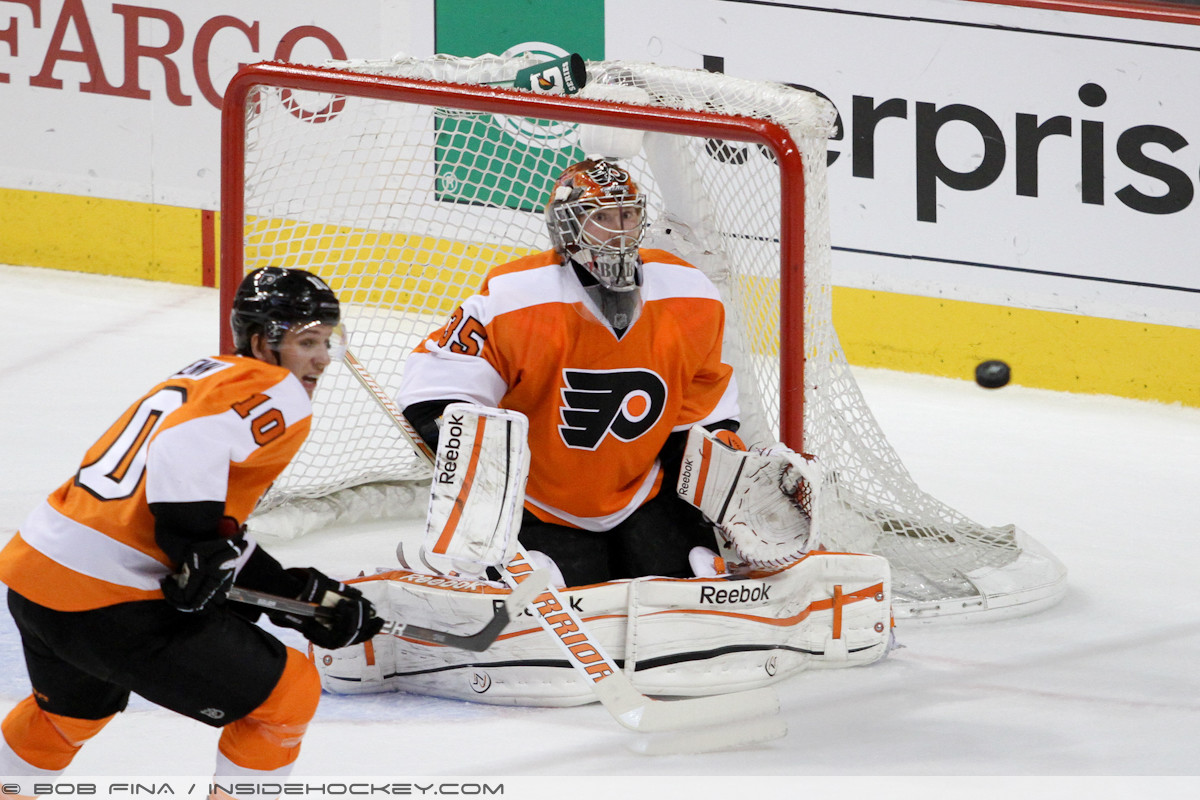The image captures an intense moment during a hockey game featuring two Philadelphia Flyers players. Central to the shot is the goalie, clad in an elaborate mask and the team's distinctive orange jersey with the prominent "P" logo and white stripes across the shoulders. The goalie is depicted making a crucial save, with his pads flattened on the ice, his glove down to his left, and his right hand gripping the hockey stick. In front of him, the puck is visible against the yellow bottom of the boards, caught in mid-air. The net behind the goalie has a red frame and looms as a stark backdrop to the action. Also in the frame is a teammate, number 10, positioned to the left. He appears focused on the puck, his stick gripped in both hands and his mouth open, suggesting exertion. The boards in the background are festooned with advertisements, adding to the dynamic atmosphere of the scene.